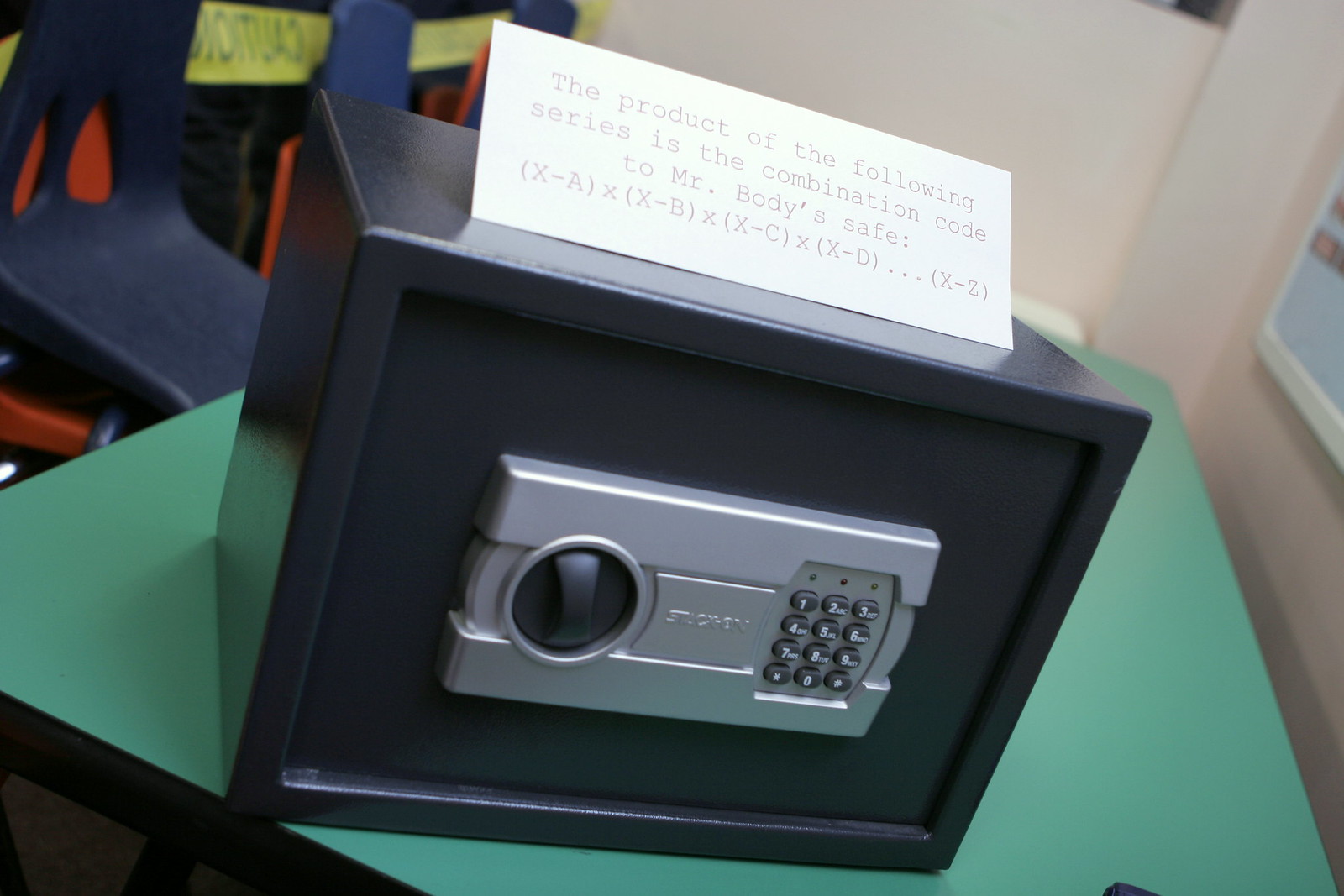In the photograph, a rectangular black safe is prominently displayed on a green table situated in the corner of a white-walled room. To the right of the table, a blue chair is pulled up close, facing the safe. The safe features a silver control panel on the front, equipped with a black knob and a keypad that includes white numbers 1 through 9, a zero, and various symbols such as a number sign and an asterisk. Though the brand name on the safe is visible, it remains illegible. 

Perched atop the safe is a white piece of paper, arranged in a tent style, bearing a message in a tight black font: "The product of the following series is the combination code to Mr. Body's safe. (x - a)(x - b)(x - c)(x - d)...(x - z)." This cryptic note suggests a mathematical puzzle, possibly hinting at the safe’s combination code, giving the scene an air of puzzle-solving or an educational setting.

In the room's background, a corner of the white wall is visible, and there are additional chairs in various colors -- red, yellow, and blue -- further enhancing the colorful yet clean atmosphere of the setting. This detailed scene conjures up thoughts of an escape room scenario or a math classroom with an intriguing puzzle to solve.